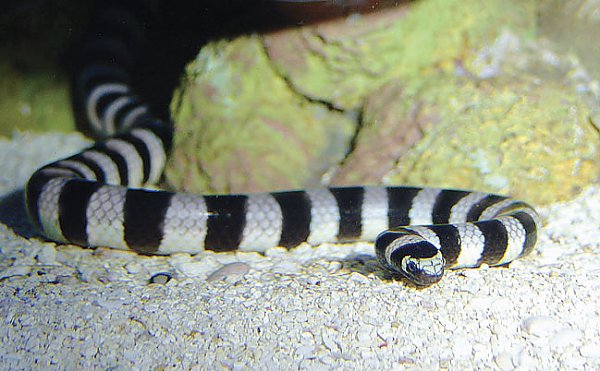This image showcases a black and white striped snake, reminiscent of a zebra's pattern, positioned on a bed of gray and white gravel. The snake's body curves gracefully, with its head oriented toward the camera and slightly towards the bottom right corner of the frame. The face of the snake is predominantly white with distinct black markings around its eyes and noseband. The backdrop features a prominent green, brown, and white mottled rock formation, occupying a significant portion of the image, mostly on the left side. The scene's precise location is ambiguous, whether it’s within a container or in the wild, but the frame is predominantly focused on the snake surrounded by its rocky environment, giving it a coiling appearance as it maneuvers around the rock. The top right corner of the image is almost entirely black, possibly hinting at shadow or the edge of the container.